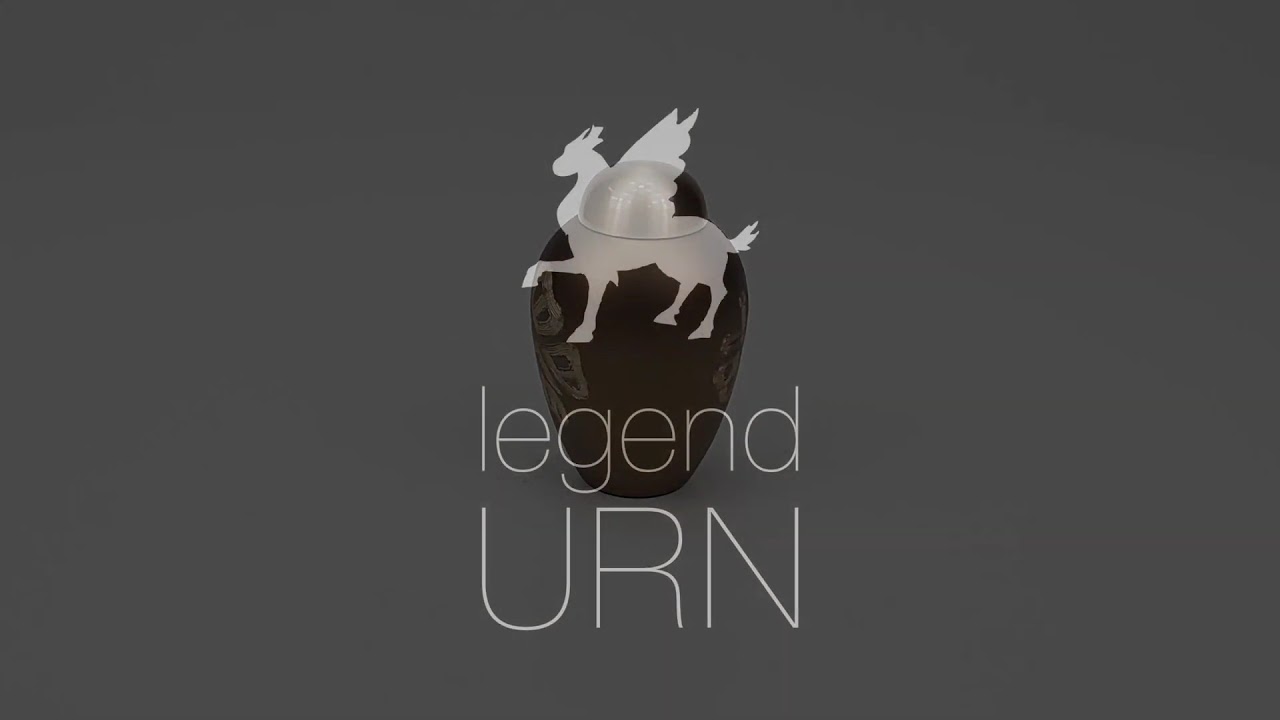The image is a detailed advertisement for an urn, featuring a dark bronze urn prominently centered against a charcoal gray background. The urn, with its semi-spherical dome cap, is adorned with intricate white flower patterns along its edges and casts a subtle shadow on the abstract gray surface beneath it. Superimposed above the urn is a white outline graphic of a mythical creature resembling a griffin, blending characteristics of a horse's body, a lion's head, and wings. Below this, in thin white text, "LEGEND" is written in lowercase, and "URN" in uppercase letters, both in a delicate, slender font. The overall design suggests a sophisticated and somber mood, suitable for a company specializing in urns.